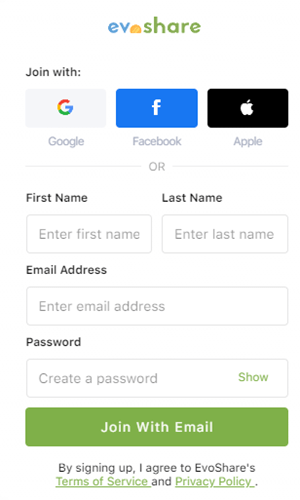A screenshot of the EV Share website's sign-up page is displayed. The header features the text "EV Share," with "EV" in blue and "Share" in green, separated by an orange icon. The interface offers four sign-up options: Google, Facebook, Apple, or manual entry. For manual entry, fields are provided for first name, last name, email address, and password, with an option to show the password by clicking "show" within the password box. Below these fields, a green button with white text prompts users to "Join with Email." A disclaimer beneath the button states, "By signing up I agree to EV Share's Terms of Service and Privacy Policy," with both "Terms of Service" and "Privacy Policy" highlighted in green and clickable for further reading. The layout is clean, intuitive, and straightforward, ensuring easy navigation for new users.